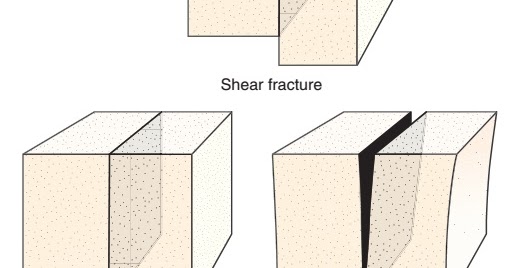The image is a detailed infographic with the title "Shear Fracture" prominently displayed in black text at the center. The visual elements consist of three groups of two rectangular, slightly translucent, cube-shaped blocks. All the rectangles have a beige color adorned with black polka dots. The background is a plain white, enhancing the simplicity of the graphic.

In the top group, only the bottom part of the rectangles is visible. The middle and bottom groups show the top three-quarters of the rectangles, creating an overlapping visual effect. The blocks are arranged in two tiers at the bottom, with the left pair positioned side by side and the right pair slightly separated to reveal a black area between them, suggesting the concept of shear fracture. The sides of the translucent blocks reveal some visual depth, especially on the right side, emphasizing their 3D nature. Minor pink and light blue shading add a subtle texture to the otherwise minimalistic design.